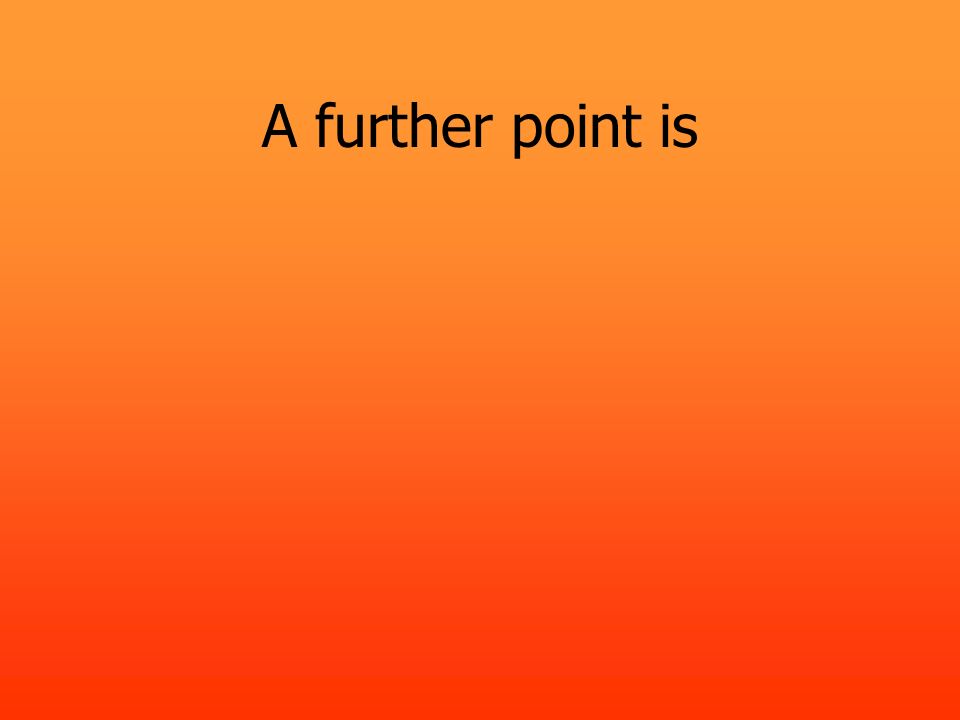The image features a square digitally created background that transitions smoothly from a light orange at the top to a darker pinkish-orange at the bottom, resembling a tropical sunset. Centrally placed towards the top of this gradient background is a line of text in black, stating "A further point is." The text consists of a capital "A" followed by lowercase letters, and occupies about the top 20-25% of the image. The rest of the image showcases the uninterrupted gradient color, providing a blank space that contrasts with the centrally placed text.